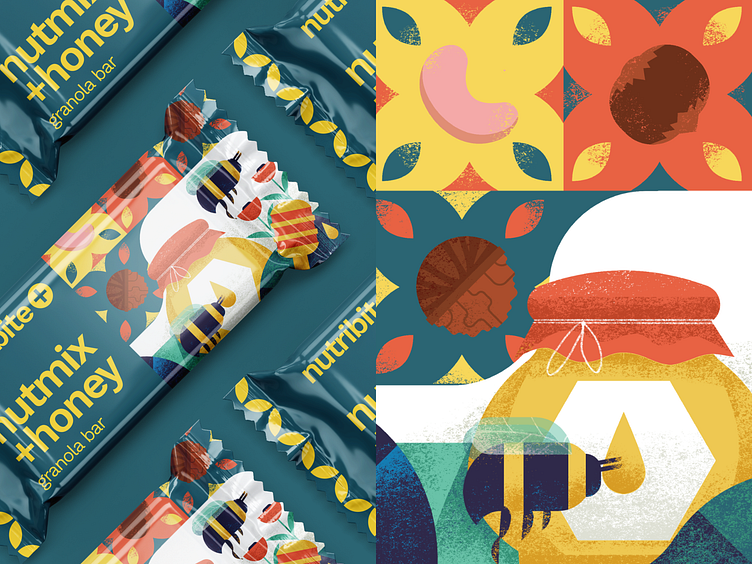The advertisement image for NutriBit's "Nut Mix Plus Honey" granola bars features a highly stylized and visually appealing design. The left half of the image displays a grid of granola bars arranged at a 45-degree angle, packaged in dark emerald green wrappers adorned with geometric illustrations. These wrappers reflect the detailed artwork present on the right half of the image, which is split into two main sections.

The right top portion showcases various types of nuts, including what appears to be cashews and other unspecified nuts, set against a vibrant background. This section is divided into a yellow left side interspersed with blue and red accents, and a reddish right side with blue and yellow accents. Beneath this, a digitally drawn bee is seen hovering near a honey jar wrapped in a red cloth with white string, placed on a white background embellished with blue and green designs.

The packaging also features a circular logo with a plus sign, rendered in warm yellow, that reads "NutriBit." The comprehensive visual makeup incorporates a mix of yellow, blue, and orangey red colors to create a cohesive and eye-catching geometric look. The detailed component illustrations on the wrappers, now blown up on the right side of the image, emphasize the nourishing blend of nuts and honey in the granola bars, ensuring the brand’s message of wholesome and easy-to-open snacks is clearly conveyed.